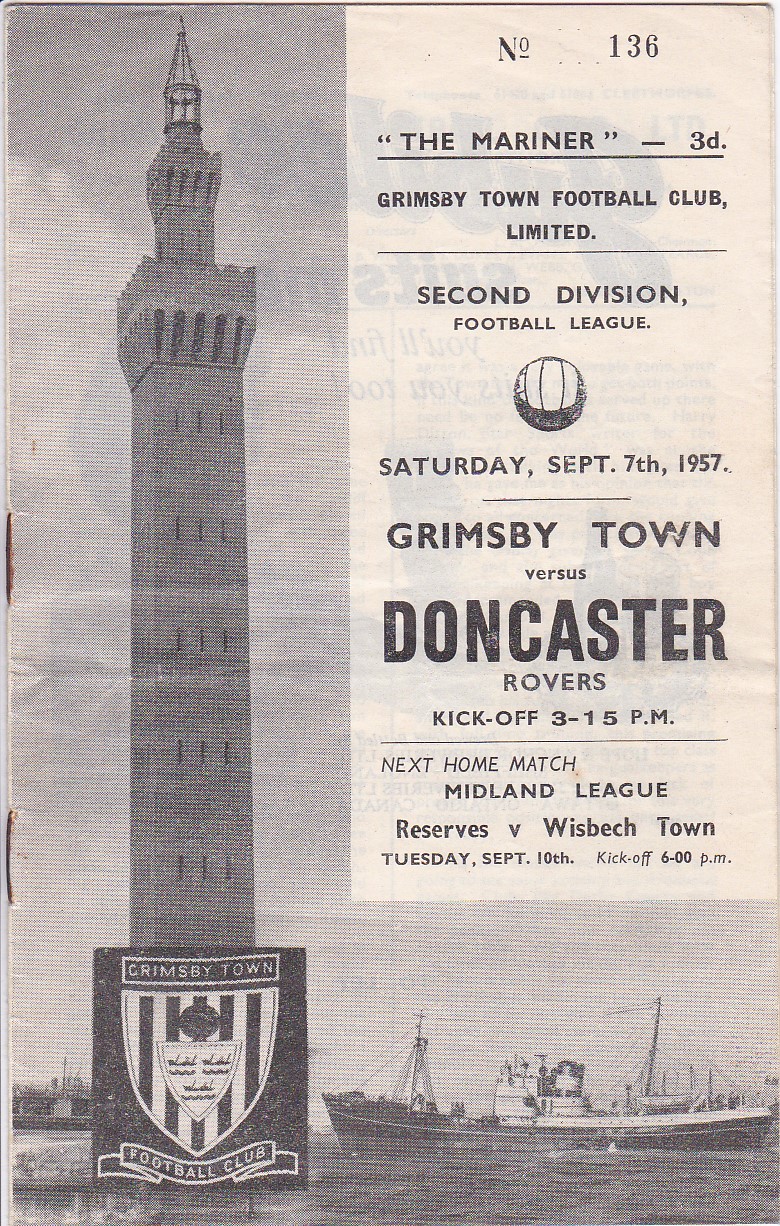This is an image of a vintage ticket for a sporting event, specifically a football (soccer) match. The ticket, dated Saturday, September 7th, 1957, is heavily detailed with both text and illustrations. At the very top, it displays "No. 136" in an old-style font, resembling "N O 136." Below this, in quotes, it reads "The Mariner / 3D," followed by "Grimsby Town Football Club Limited" in a bold print, indicating the hosting team. The event is categorized under the "Second Division Football League."

There is a prominently handwritten illustration of a football (soccer ball) on the ticket. The main event details, rendered in heavier print, note that the match will feature "Grimsby Town vs. Doncaster Rovers," with the kickoff scheduled for 3:15 PM. Below this are details of the next home match against "Wisbech Town," which is scheduled for Tuesday, September 10th, with a 6:00 PM kickoff. This upcoming match is part of the "Midland League" reserves.

The background of the ticket features intricate, monochrome illustrations. On the left side, a very tall tower dominates the scene, with a banner at its base bearing a shield. Surrounding the tower is water with a ship traversing it. Above and behind the tower, clouds fill the sky, all rendered in deep gray, black, and white tones, providing a vintage and historic feel to the ticket. The combination of detailed textual and graphic elements gives this ticket a rich, nostalgic character, representative of mid-20th century football culture.